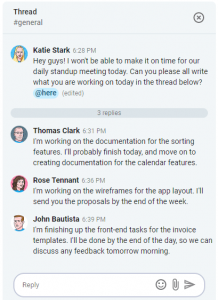The image displays a text conversation set against a very light gray background, presented in a slightly vertical orientation. The conversation features contributions from Katie Stark, Thomas Clark, Rose Tennant, and John Bautista. At the top left corner, a label reads "Thread #general."

Each participant is represented by a colored circular icon to the left of their name. Katie Stark initiates the thread with the original post, which reads: 

"Hey guys, I won't be able to make it on time for our daily standup meeting today. Can you all please write what you are working on today in the thread below? @here."

The "@here" tag is outlined in light blue. Below Katie's message, a thin gray bar indicates that there are "3 replies."

The subsequent replies follow in chronological order:

- Thomas Clark at 6:31 PM: "I'm working on the documentation for the sorting features. I will probably finish today and move on to creating documentation for the calendar features."
- Rose Tennant at 6:36 PM: "I'm working on the wireframes for the app layout. I'll send you the proposals by the end of the week."
- John Bautista at 6:39 PM: "I'm finishing up the front-end tasks for the invoice templates. I'll be done by the end of the day so we can discuss any feedback tomorrow morning."

At the bottom of the image, there is a reply bar featuring three icons, inviting further interaction.